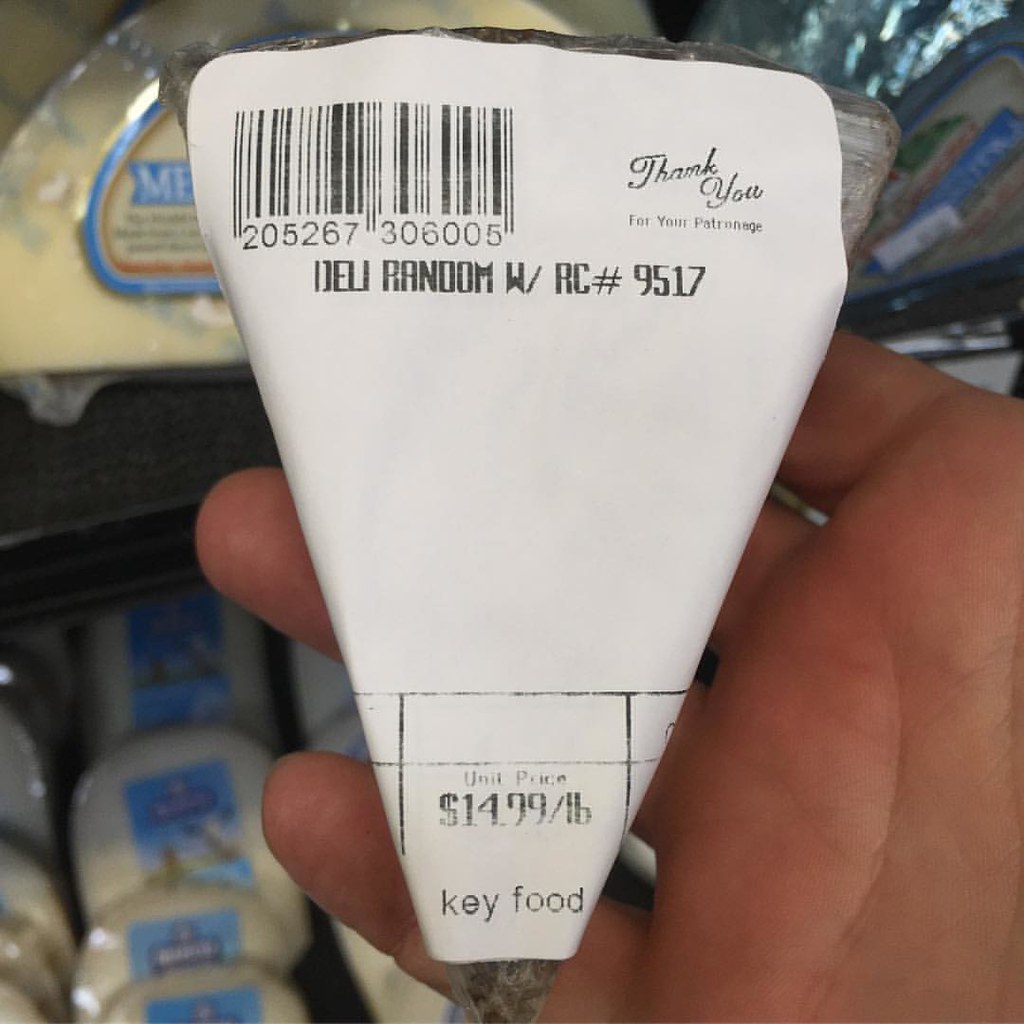The image depicts a triangular wedge of deli item, likely cheese, wrapped in crisp white paper. The paper features black text with detailed information. Prominently displayed on the top left corner is a barcode with numbers 205267306005. Below the barcode, the label reads “Deli Random W/RC number 9517.” Additionally, the package includes a note of appreciation with “thank you for your patronage.” At the bottom, it lists the unit price as $14.99 per pound and identifies the brand as Key Food. The food item is being held by a person, capturing a close-up photograph, with a background showing various colorful cheeses on a shelf, many of which are in clear packaging adorned with blue text.